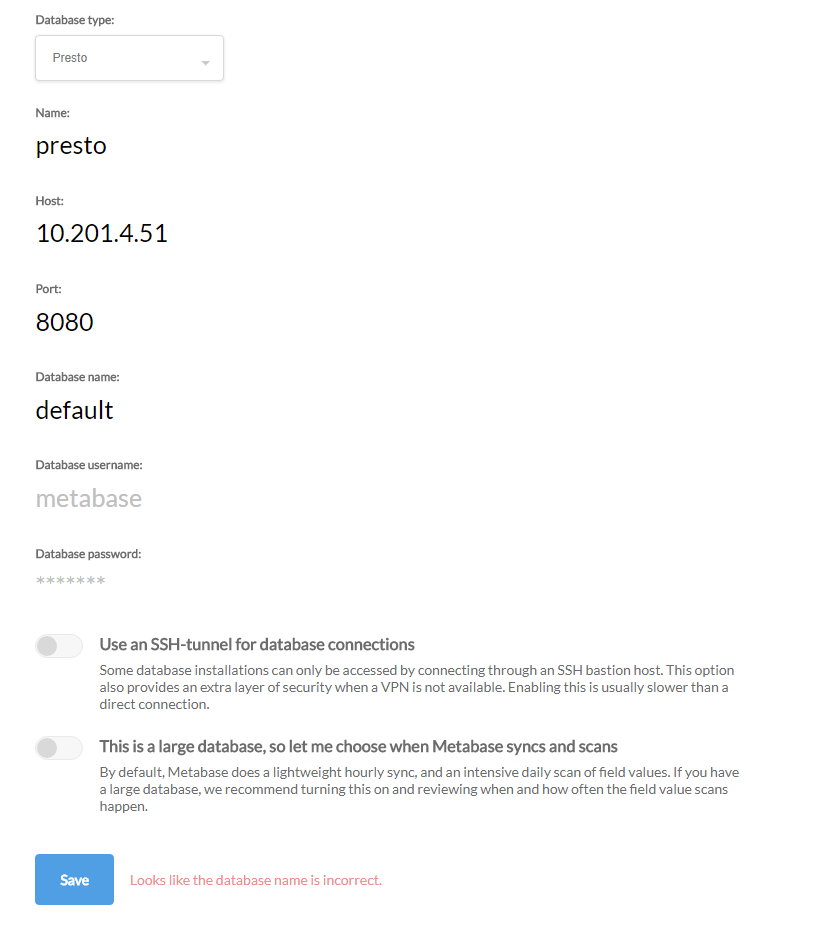The image is a screenshot of a database configuration interface set against a solid white background. In the top left corner, small black text reads "Database Type." Below this, there is a white dropdown button labeled "Presto." Underneath the dropdown, the label "Name" appears with the text "Presto" in larger black font. Following this, the label "Host" is displayed in small text above a larger black text displaying the IP address "10.201.4.51."

Further down, the label "Port" appears above the port number "8080." Below the port, the label "Database Name" is present with the text "default" written in larger font beneath it. Following this, the label "Database Username" appears, showing the username "MetaBase" in larger text below it. The label "Database Password" is also displayed without an accompanying password.

Toward the bottom, there are two toggles that are currently not activated. The first toggle is labeled "Use an SSH tunnel for database connections," and the second toggle reads "This is a large database, so let me choose when Metabase syncs and scans."

In the lower left corner of the interface, a prominent blue "Save" button is situated.